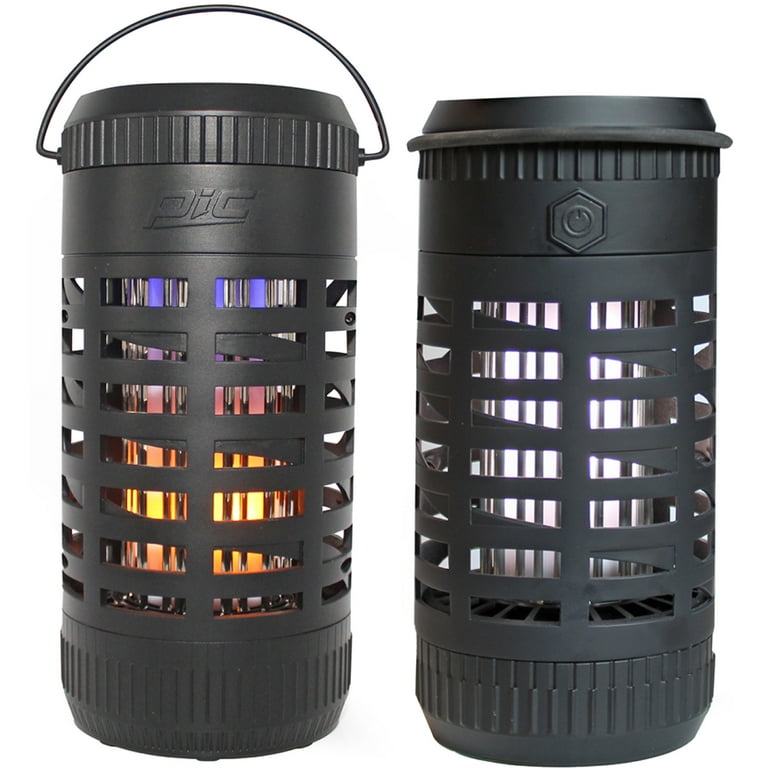The image showcases both the front and back views of a cylindrical, portable heater or heating lantern by the brand PIC. The device is predominantly black or dark gray, featuring a thin gray wire handle across the top for easy portability. The heater has a modern, sleek, and potentially battery-operated design. The front view of the heater reveals a series of weaved slats or grates in the middle section, allowing visibility of the internal heating element. This element is actively glowing in the front view, displaying vivid colors like blue, pink, orange, red, and yellow, indicating it is turned on. Raised lettering "PIC" is prominent just below the top lid on the front side, and beneath it is a small line cut into the surface. The back view, shown separately, highlights a power button symbolized by a diamond with a center dot and reveals that the internal area is not illuminated, showing a white interior or background. This detailed design ensures safety by preventing direct contact with the heating element through the exterior grate.